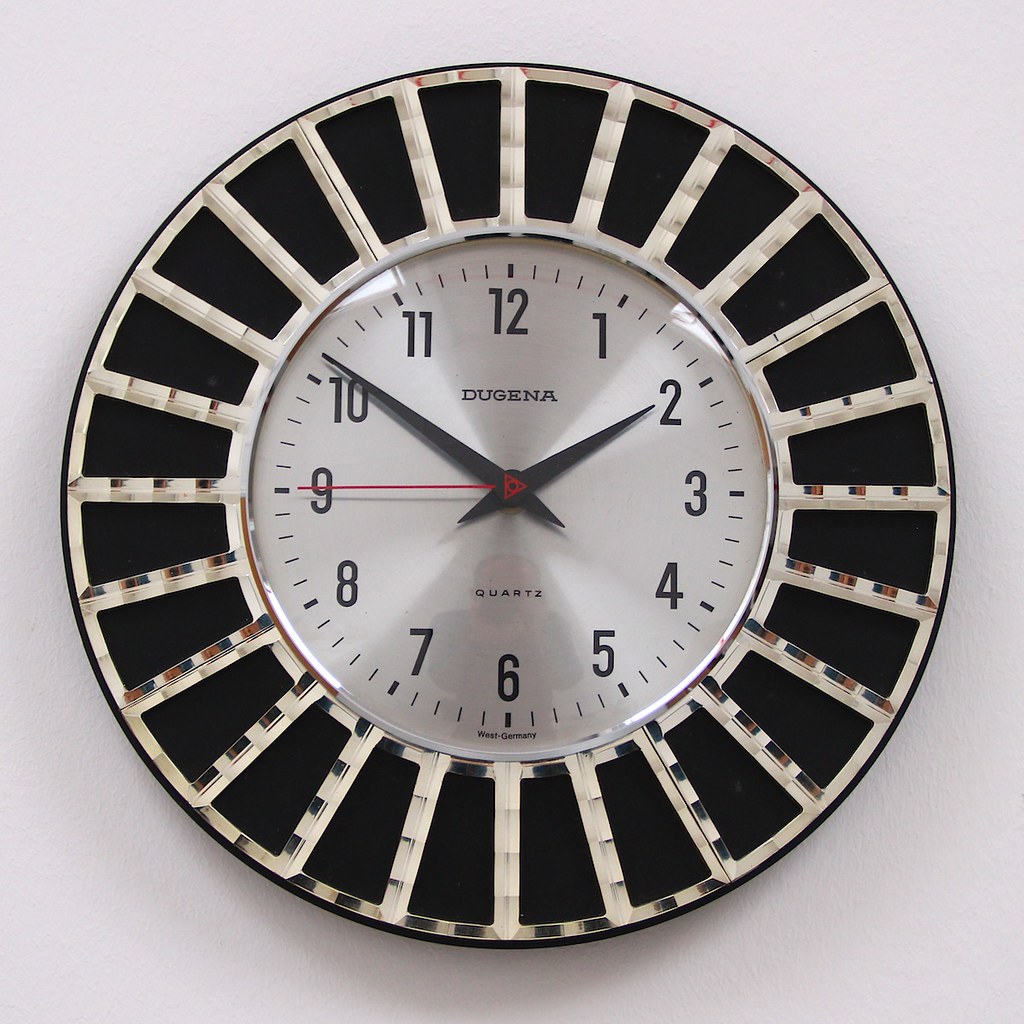This photo features a distinctive Dugena-branded clock hanging on a light gray wall. The clock has a unique design with a thick, round border comprised of alternating black and silver spokes, creating a striking visual effect. The black sections are wider towards the outer edge, giving them a stripe-like appearance. The clock's white face contrasts sharply with its black hour and minute hands, while the red second hand adds a pop of color. The time displayed is approximately 2:51, with the second hand pointing towards the 9. The clock face is marked by regular digits from 1 through 12, along with additional second markers. Above the clock hands is the brand name "Dugena," and below it reads "quartz." Notably, the reflection of the person taking the picture is faintly visible at the bottom of the clock.